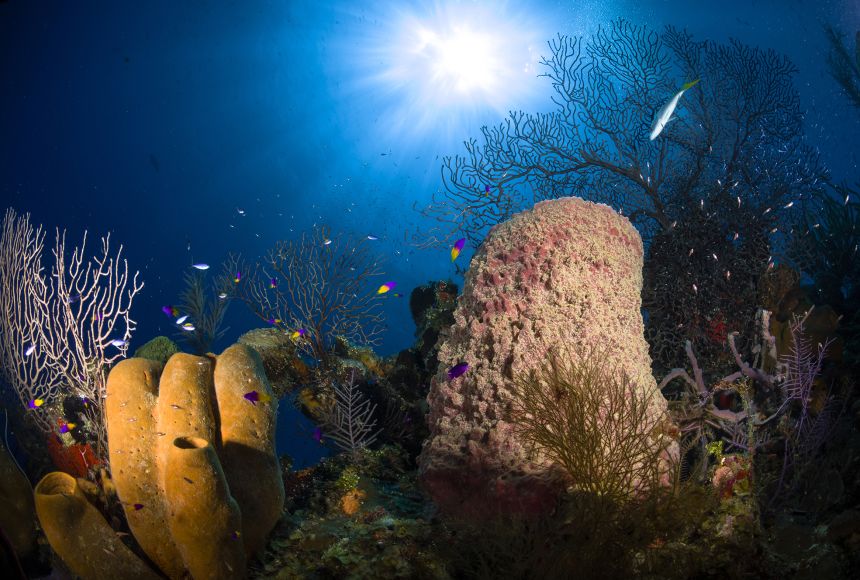The underwater photograph showcases a vibrant coral reef teeming with life. In the foreground to the left, there is a slender, light purple coral structure resembling a skinny branch. Adjacent to it is a more robust, buoyant yellow coral, and nearby, a larger coral that has a crusty texture with varying shades of light and dark pink. In the top right of the image, a longer fish with a green tail and light blue body swims downward. Various fish populate the scene, including small, electric-looking light blue fish and several purple fish, some of which are half purple and half yellow. The background is rich with more coral structures, some resembling tree branches covered in moss. Sunlight or moonlight filters down from above, illuminating the serene and flourishing underwater ecosystem.